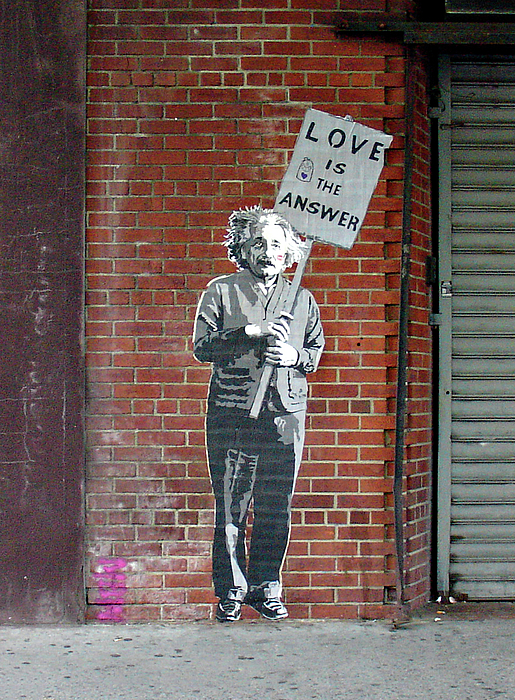This image features a striking black and white mural of Albert Einstein painted on a red brick wall. Einstein, with his iconic wild hair and mustache, faces the camera, exuding a contemplative expression accentuated with lipstick marks on his cheek. He wears a grayish cardigan buttoned up over a shirt, paired with loose dress pants and black shoes. His arms, bent at the elbows, hold a wooden pole that crosses his body and extends above his shoulder, ending in a white sign that declares in bold black letters, "Love is the Answer." The mural, illustrating Einstein holding the sign, also includes a small cartoon character with a heart on its chest smiling from within the sign. To the right of the mural, there is a dirty gray sidewalk and a white garage door partially visible. The brick wall itself is marked with some white and pink paint, adding to the gritty urban feel of the scene.